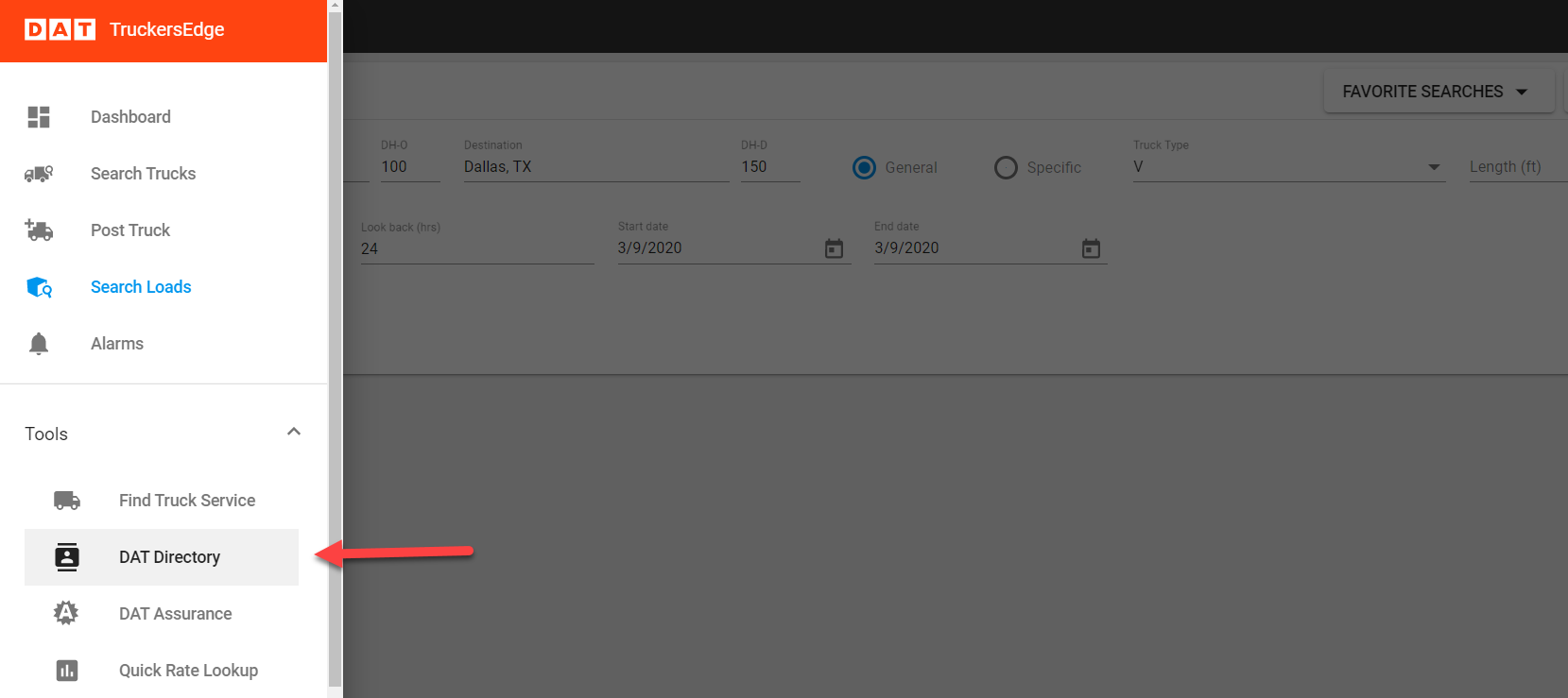The image showcases an interface from DAT Trucker's Edge. In the top left corner, there is a green rectangle with the text "DAT Trucker's Edge" displayed prominently. Below this, a vertical column lists several options in the following order: "Dashboard," "Search Trucks," and "Post Truck," followed by "Search Loads" in blue. Beneath "Search Loads," "Alarm" is displayed in black. A light gray line separates this section from the "Tools" heading below it. Under "Tools," options include "Find Truck Service" with an icon of a delivery van next to it, and "DAT Directory" which is highlighted with a gray rectangle and has a red arrow pointing towards it. Following this, "DAT Assurance" and "Quick Rate Lookup" are listed. 

To the right of this column, there's a gray scroll bar for navigation. Adjacent to the scroll bar, the main content area features an image with a gray tint, making it appear blurry and out of focus. At the top, a sleek black border frames the interface, and on the upper right side, there's a drop-down menu labeled "Favorite Searches." Below this drop-down menu, there's another, albeit darker, menu whose contents are indistinguishable due to poor visibility.